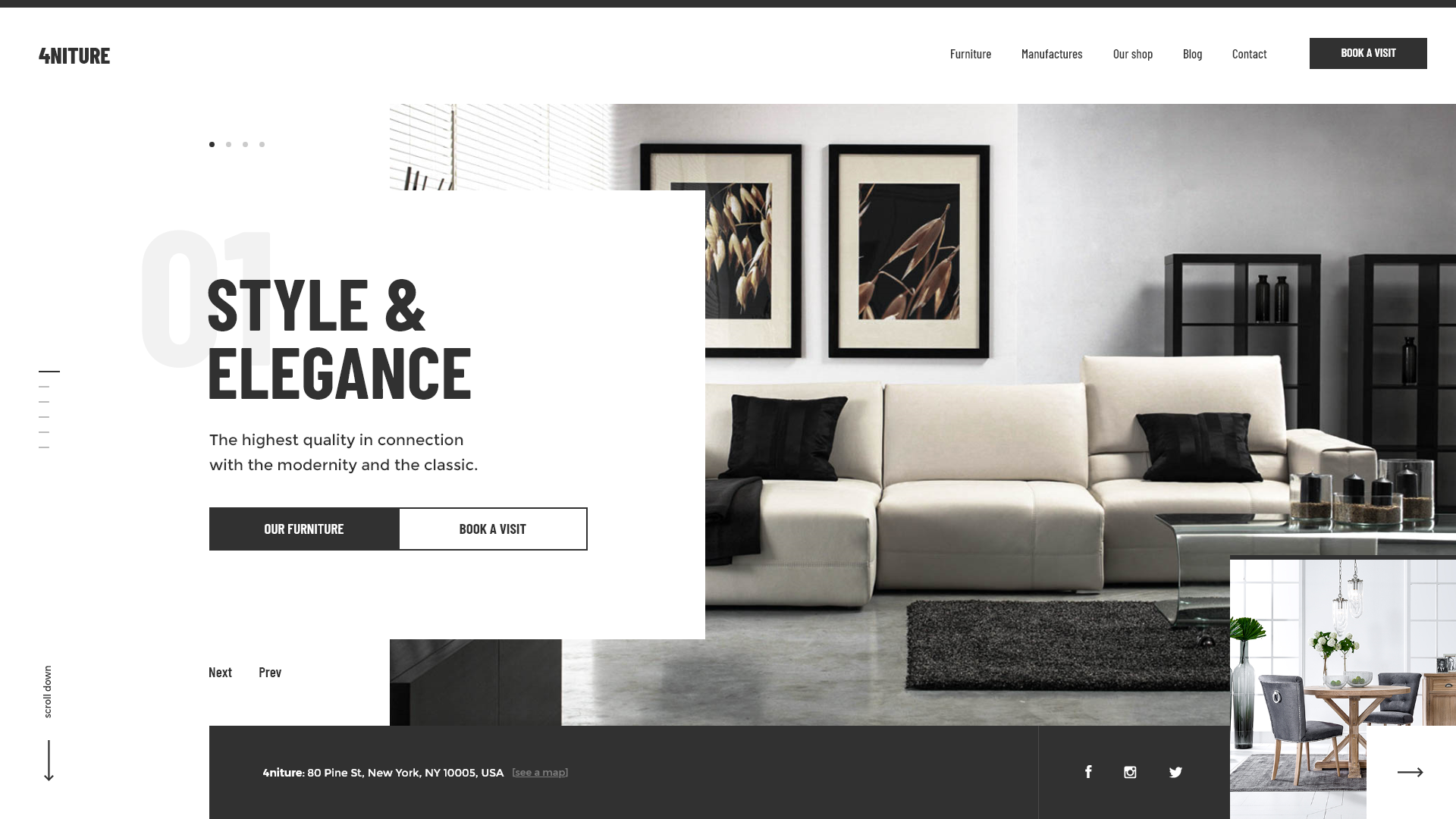This advertisement from the company "4NITURE" showcases their unique brand name prominently displayed in the upper left-hand corner of the image. The setting features a serene and calming ambiance with a palette of soft, understated colors. The background boasts a tranquil, not-too-bright scheme that enhances the room's relaxing atmosphere.

The room is furnished with a modern beige sofa, which appears mechanically adjustable, offering personalized comfort. Adorning the walls are elegant pieces of artwork in shades of beige and black. Centrally placed is a stylish glass table accompanied by a sleek black rug. The room's marble flooring adds a touch of luxury, while black shelves in the background hold small vases, adding a subtle decorative touch.

In the bottom right-hand corner, a wooden table setting is elegantly arranged with a tall vase, hanging lights from the ceiling, flowers, and bowls, all contributing to the room's contemporary aesthetic. The overall brightness of the space, predominantly white, amplifies its airy and modern feel.

"4NITURE" combines high-quality modern design with classic elements, offering a sophisticated selection of furniture. The company, based in New York, invites customers to book a visit to their showroom. They maintain an online presence on social media platforms like Facebook and Twitter and provide additional resources such as a blog, contact information, and an option to book a visit on their website.